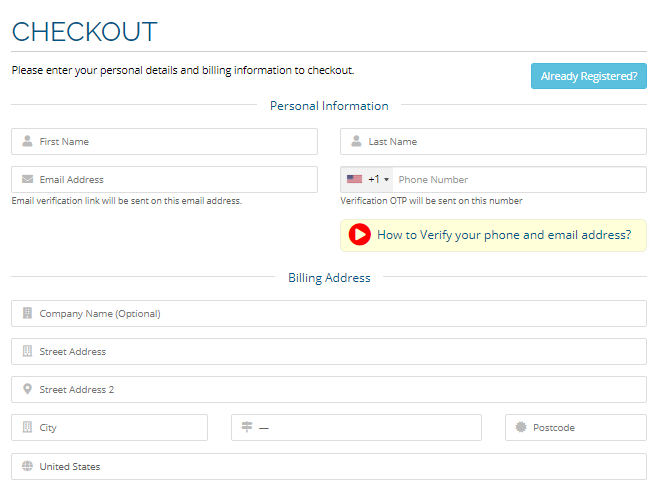The image showcases a detailed checkout form designed for users to enter their personal and billing information. The form includes several fields: a blue square button labeled "R" for registration, a question mark icon, and sections for personal information such as first name, last name, email address, telephone number, and email verification. An email verification link will be sent to the provided email address, and an SMS verification code (LTP) will be sent to the phone number.

There is also a "Play" button, followed by instructions on how to verify the phone number and email address. The form contains sections for billing information, including billing address lines, an optional company name field, a street address field marked by a pin icon, a secondary street address field, a city field with an icon resembling a sign board, a postal code field, and a dropdown for selecting the country, which in this case shows "United States." The top left and bottom right sections of the image are gray, contrasting with the predominantly white background, and the form is visually segmented by various lines and dividers to organize the information fields clearly.